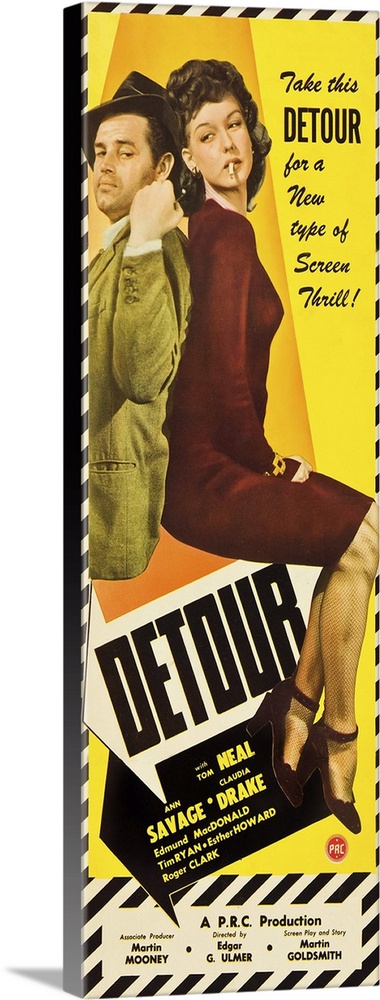This image is an old-fashioned movie poster from the 1940s advertising the film "Detour." The poster is tall and thin, framed by a black and white striped border with a yellow background. Featured prominently are a man and a woman sitting back-to-back, seemingly on a sign. The man, wearing an old-fashioned hat and a greenish-white collared shirt, looks over his shoulder at the woman. She has curly brown hair, a cigarette in her mouth, and wears a burgundy-colored dress with matching shoes. The tagline "Take this detour for a new type of screen thrill" appears on the right side of the poster. Below them, two large arrows, one white with big black letters spelling "Detour" and the other black, list the actors as Tom Neill, Ann Savage, Claudia Drake, Edmund MacDonald, Tom Ryan, Esther Howard, and Roger Clark. The poster also credits director Edgar G. Ulmer, screenplay writer Martin Goldsmith, and associate producer Martin Mooney, marking it as a PRC production.